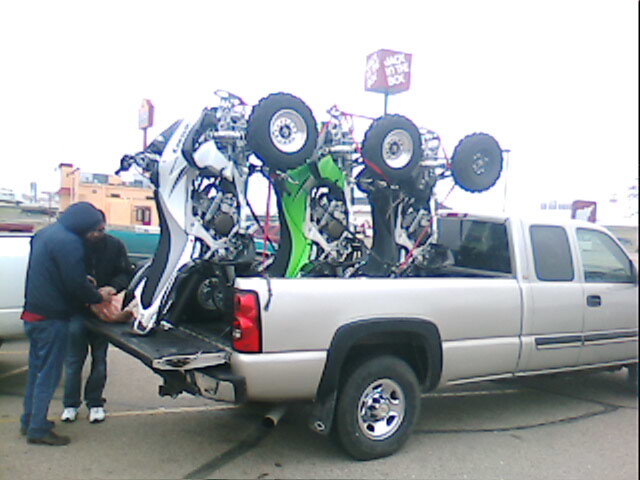In an outdoor setting with a cloudy sky, a medium gray pickup truck, featuring black plastic wheel wells, stands parked in a lot. The tailgate is open, revealing three four-wheeler ATVs stacked vertically and secured with nylon straps: a white one with a black seat, a green one in the center, and a black one. Two men are standing nearby, seemingly working on or attending to the ATVs. One man is dressed in black pants and a black sweater, while the other wears jeans, work boots, a blue sweatshirt with the hood up, and a red shirt peeking out from underneath. In the background, several buildings are visible, including a Taco Bell and a Jack in the Box, with distinct signage marking each location. The overcast condition creates a soft shadow beneath the truck, emphasizing the gray ambiance of the day.